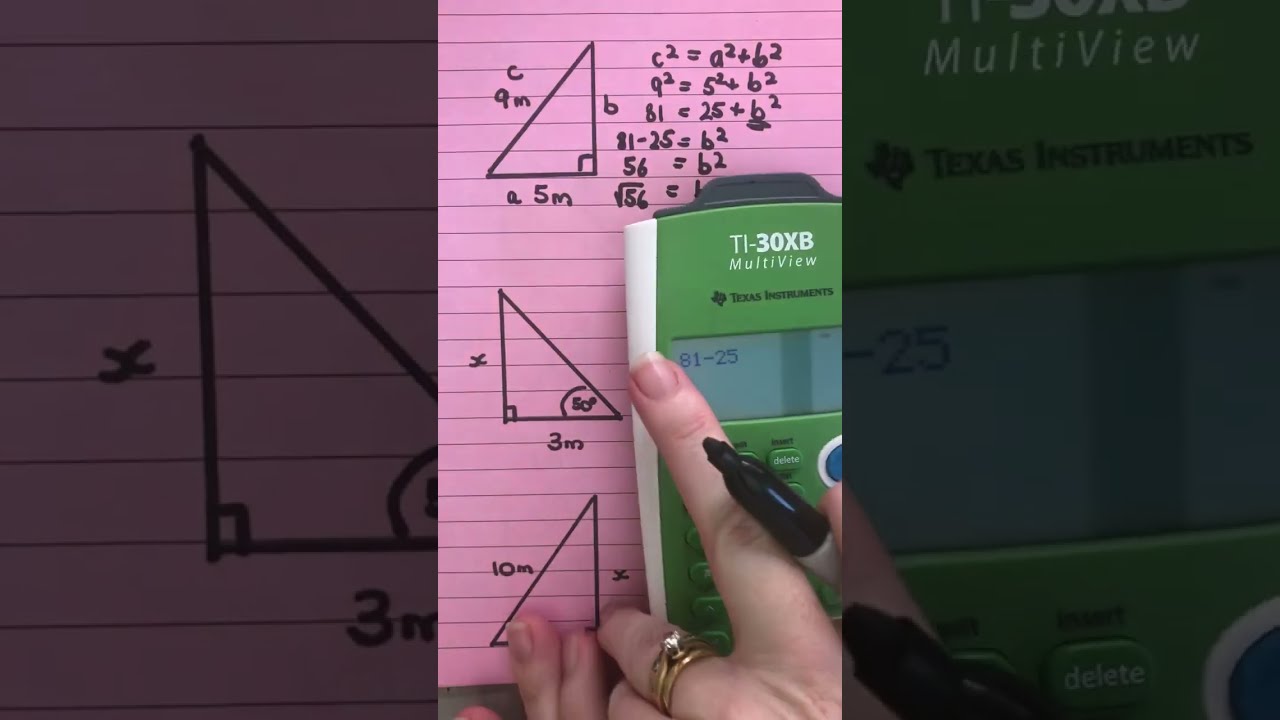A detailed image captures a vibrant scene of geometry homework on a purple/pink college-ruled paper. Dominating the center is a neatly written breakdown of equations and translations related to right-angled triangles, thoroughly showcasing formulas and measurements. In the bottom right corner sits a green TI-30XB MultiView scientific calculator by Texas Instruments, actively engaged in calculations, displaying "01-25." The focal image is flanked by zoomed-in, faded versions of itself, creating a distinctive border. A woman's hands, emerging from the bottom of the image, demonstrate precise work with a black Sharpie marker in her right hand. Her left hand, adorned with a wedding band and an engagement ring featuring a single solitaire diamond, steadies the paper and cradles the calculator. The entire setup highlights her meticulous approach to solving the math problems.